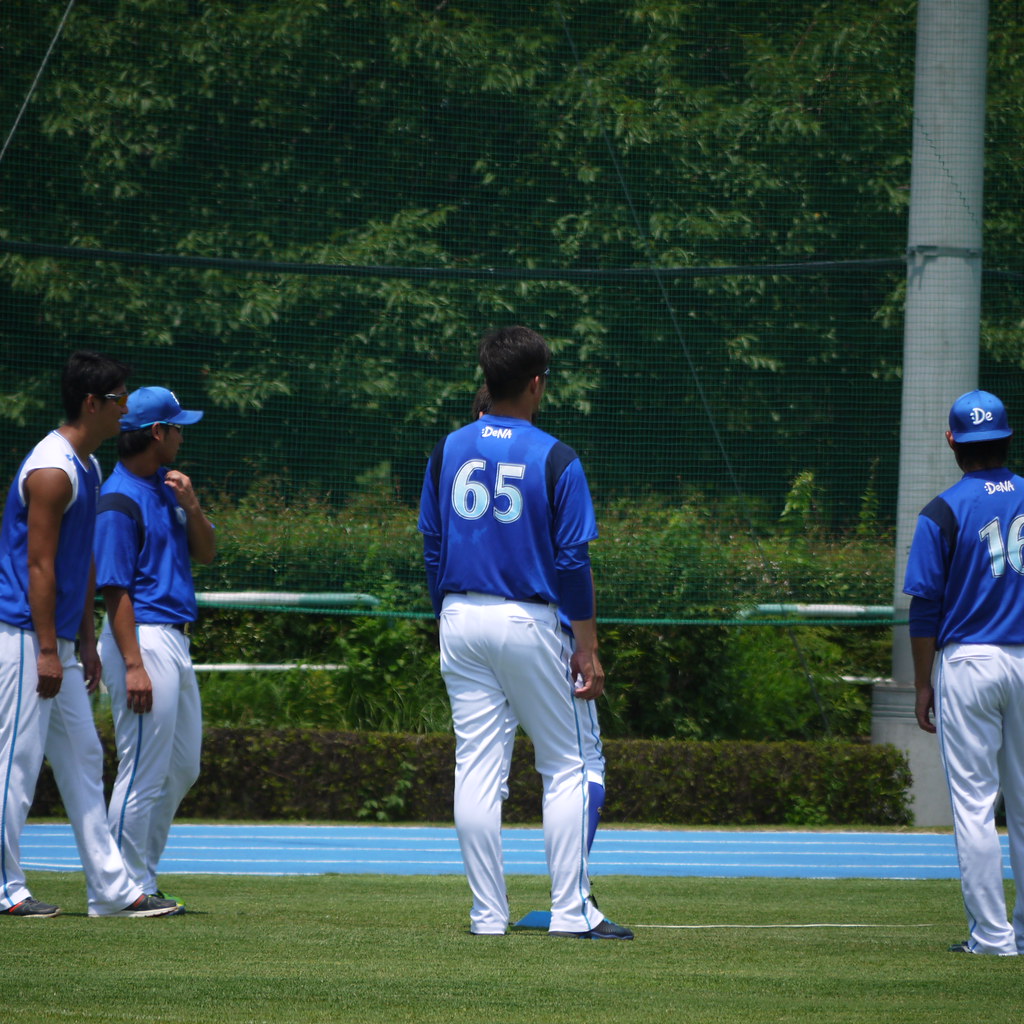This is a detailed outdoor photograph taken during a daytime track and field event, cropped into a square shape. The image features a team of young boys, likely in high school, all with darker skin tones and black hair, standing on short-cut green grass. They are all uniformly dressed in white long pants with a blue pinstripe down the left side and blue short-sleeved jerseys with navy blue bands at the shoulders and white numbers on the back. The boy in front has the number 65 and an unreadable word at the top of his jersey. Some boys wear dark long-sleeved shirts under their jerseys, while one boy on the far left has a sleeveless jersey with white and blue colors. Several boys sport blue baseball caps, worn backwards. They are facing a tall black mesh net, resembling a volleyball net, and are either waiting for a game to start, discussing a strategy, or watching an ongoing event. Behind the net lies a four-lane running track, and further beyond, the landscape transitions from small shrubs, to taller bushes, and finally a line of tall trees. The bottom fifth of the photo focuses on the vivid green grass, and a small blue ball, about the size of a baseball, rests on the ground, adding an element of uncertainty regarding the sport.